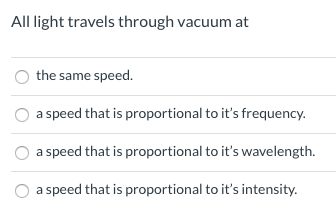This square-shaped image features black text set against a white background, accompanied by gray lines and circular bullet points. At the top of the image, the text reads, "All light travels through vacuum at." Below this phrase, a horizontal gray line spans the width of the image, dividing the header from the listed statements. Each statement is prefaced by a circular, gray bullet point aligned on the left side. The sequential bullet points contain the following text:

1. The same speed
2. A speed that is proportional to its frequency
3. A speed that is proportional to its wavelength
4. A speed that is proportional to its intensity

The overall minimalist design emphasizes clarity, with the primary visual elements being the black text, gray dividing lines, and the structured arrangement of bullet points on a crisp, white background.